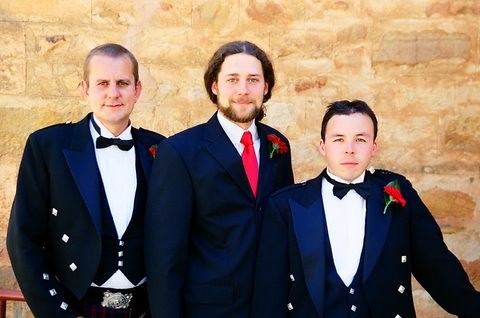The image depicts three formally dressed men standing outside against a large, stone wall with a mix of vanilla yellow, white, and dark brown hues. All three men are wearing blue suits with a sheen, displaying slight variances in the color of their lapels. Each man has a red rose pinned to their lapel.

On the left, the man is dressed in a blue jacket with slightly lighter blue lapels, a dark blue bow tie, a vest underneath, and a silver belt buckle peeking from behind another person. His attire includes diamond-shaped buttons, and he has a dark blue bow tie and dark hair.

In the middle stands a man with longer hair, a mustache, and a goatee. He is wearing a white shirt paired with a blue suit, a red tie, and a red rose. Unlike the others, his suit lacks buttons.

The man on the right, smaller than the others, is also wearing a dark blue suit with lighter blue lapels and a vest underneath. He sports a blue bow tie and dark hair, matching the formal attire of his companions, but with a similar diamond-shaped buttons detail on his suit.

A shared characteristic among them is the presence of red roses on their suits, adding a formal touch to their coordinated appearance.